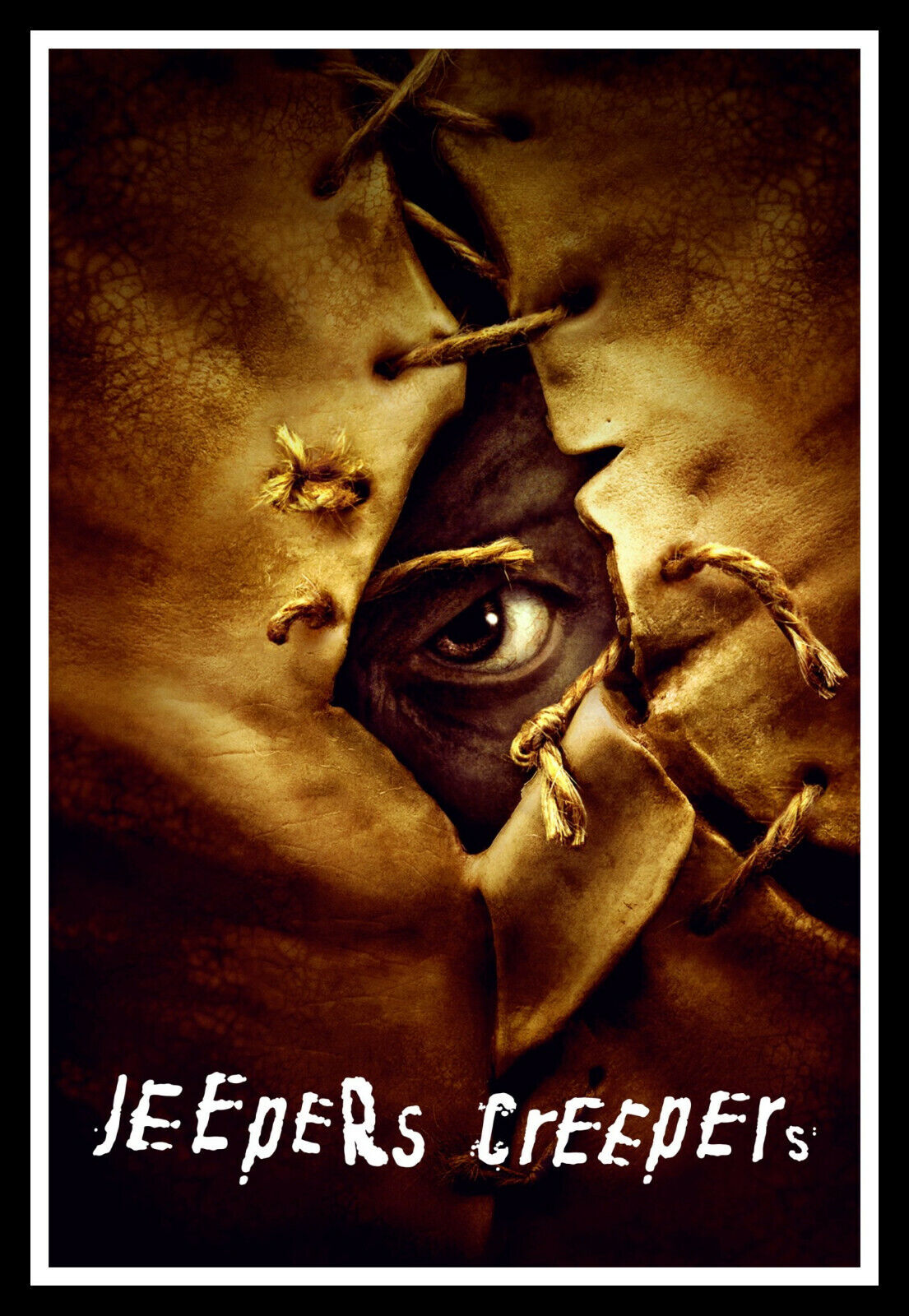This is a surrealist movie poster for "Jeepers Creepers" featuring a close-up design primarily in dark and light browns. The central image shows an eyeball peering out from a stitched-together leather or canvas bag, with the ties coming loose enough to allow the eye to be visible. The background is dark, creating a stark contrast with the light brown of the bag. The eyeball is set within a hole in the bag, looking ominous and adding a scary tone to the image. Surrounding the main image is a tall black rectangle with a white border, enhancing the eerie and mysterious feel of the poster. At the bottom, in capital letters, the white text reads "Jeepers Creepers," completing the unsettling and mysterious aesthetic of the movie poster.